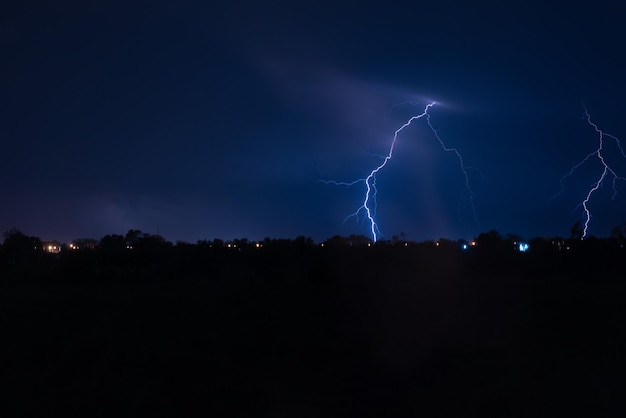This nighttime live action photo captures an atmospheric scene just after dusk. The bottom half of the image is almost completely black, silhouetting the horizon which is lined with trees and houses, some of which have their lights on, resembling tiny white dots scattered across the dark expanse. The sky above transitions to a deep, stormy blue and purple, with shadowed clouds indicating active rain in parts of the scene. Dominating the image, a vivid lightning strike mostly in the center, just off to the right, descends from the clouds to the ground, casting light that illuminates the sky in a striking blue hue. Another, less intense lightning strike is situated further to the right near the edge of the photo. The dramatic lighting provided by these bolts makes the dark stormy sky the primary focus of the image, showcasing nature's powerful energy arcs against the tranquil suburban horizon.